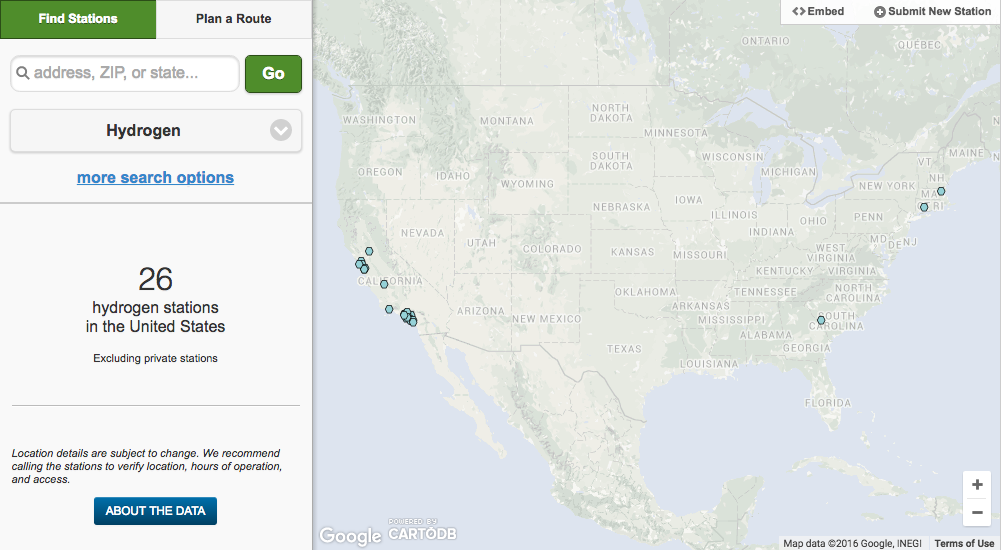The image depicts a user interface of an application designed to locate hydrogen stations, among possibly other types of fueling stations, within the United States. The central feature of the interface is a highly detailed map displaying the spread of hydrogen stations across the country. Most of the stations are indicated by blue dots concentrated in California, particularly around the Bay Area and Southern California, with a few scattered in central California. Additionally, there are sporadic blue dots in the eastern part of the country, notably in the Carolinas, Massachusetts, and a few other states in the Northeast. The map seems to have a bleached appearance, with data imported from Google Maps, as indicated by the branding.

On the left side of the interface, there is a vertical panel for user interaction. At the top, it has an option labeled "Find Stations or Plan a Route," with "Find Stations" being selected. This selection is highlighted in solid green with white text. Directly below, there is a search field where users can input an address, ZIP code, or state to find specific locations, accompanied by a green "Go" button for initiating the search.

Further down, there's a drop-down menu labeled "Hydrogen," which suggests the possibility of selecting other types of fuel. A blue text link titled "More Search Options" sits below this menu for additional filtering choices.

The main section of this panel shows a message stating there are 26 hydrogen stations available in the United States, excluding private stations. Below this statement is a thin gray line, followed by a disclaimer advising users to verify station details by calling ahead to confirm locations, hours of operation, and accessibility.

At the bottom of the left panel is a blue rectangular button labeled "About the Data," which likely provides more information on the sources and accuracy of the displayed information. The app does not display any other branding or detailed information about additional search options, leaving some ambiguities about its full capabilities, such as whether it includes propane or gasoline stations.